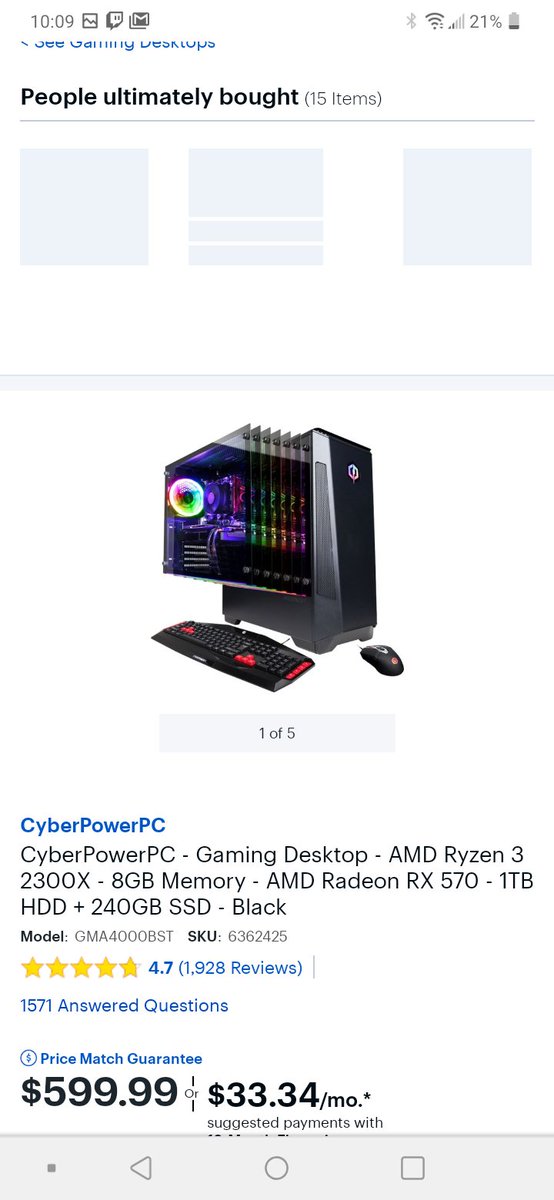Sure, here’s a well-organized and detailed caption:

---

"An image displays a CyberPowerPC gaming desktop for sale. The primary focus is on a black tower, with an additional pop-out section detailing the internal components. It's equipped with an AMD Ryzen 3 2300X processor, 8GB of memory, an AMD Radeon RX 570 graphics card, a 1TB HDD, and a 240GB SSD. The model number is GMA4000BST and the SKU is 6362425. The product has received an impressive rating of 4.7 stars from 1,928 reviews, and there are 1,571 answered questions about it. The price is listed as $599.99, with a price match guarantee, or available for $33.34 per month through suggested payment plans.

In the background, it is evident that the photo was taken on someone's phone, which is currently at 21% battery life, indicated by the Wi-Fi, cellular, Bluetooth, and email icons visible at the top of the screen. The time shown is 10:09. The product listing also notes that customers typically purchase an additional 15 items with this desktop."

---